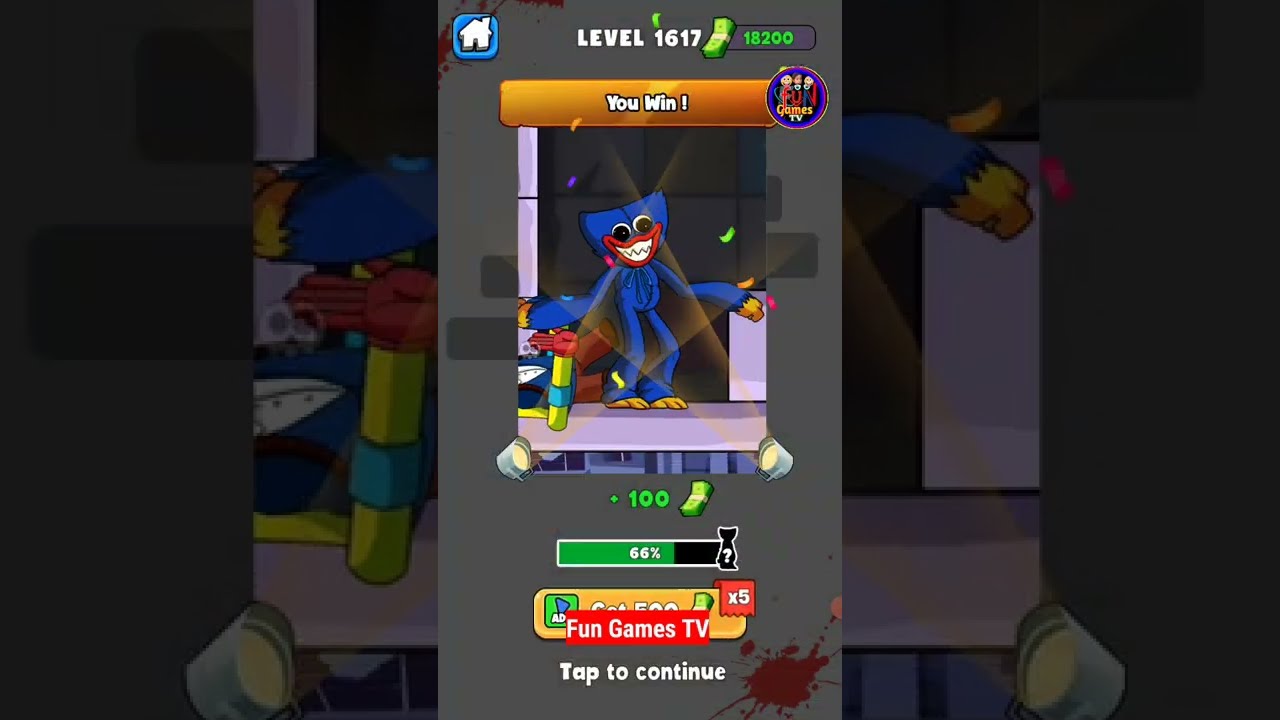This is a detailed and descriptive screenshot of a mobile game displayed on a cell phone, presented in a portrait orientation against a darkened, landscape background. Central to the image is a vividly animated blue character, possessing a mix of features that combine a distorted Elmo and Grover. This character, with large red smiling lips, a square top head, black and white eyes, long arms, and long legs, stands out vividly against a gray background that resembles a brick wall. Above the character's head, the game announces "You Win" in white script, indicating the completion of level 1617. The player has earned a notable amount of 18,200 with dollar signs next to it, although it's unclear if this represents real money. Surrounding the character are various statistics including a bar showing progress at 60%, a minus 100 next to a stack of dollar bills at the bottom, and a red banner that reads "Fun Games TV" with the directive "Tap to continue." The character seems to be in an animated or celebratory pose, adding to the eerie effect with its wide, unsettling grin and repetitive proclamation of victory, "you won, you won, you won."